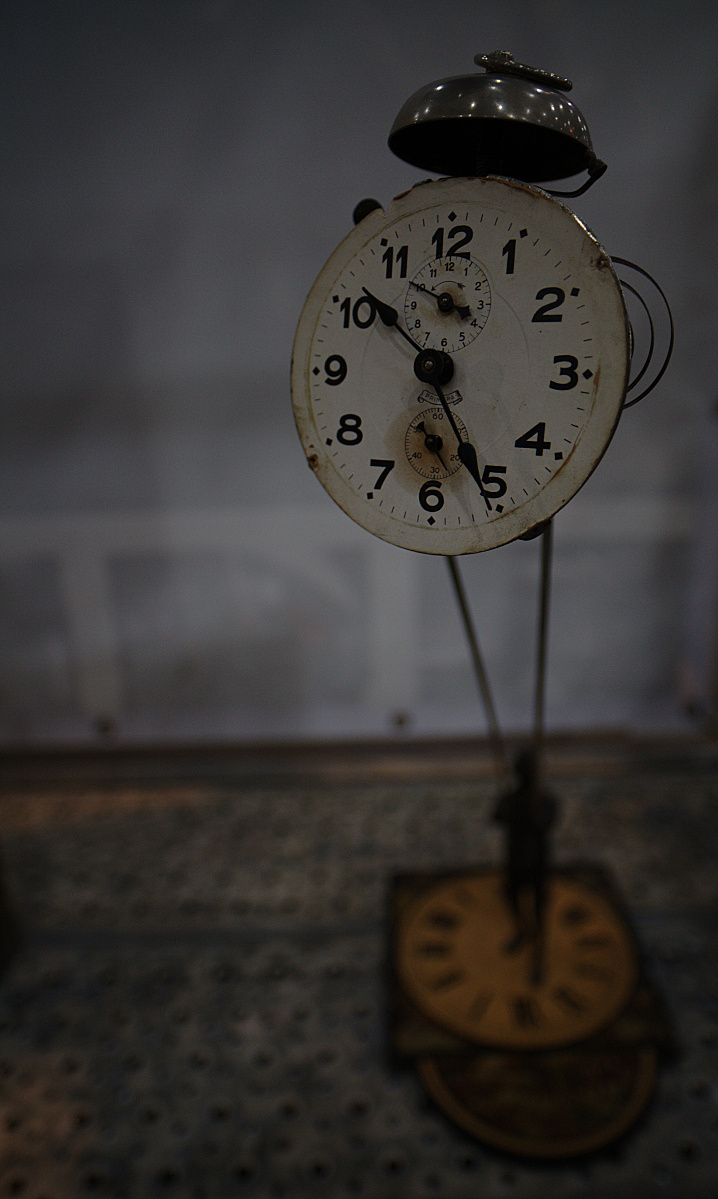This detailed indoor, low-light close-up photograph captures an artistic sculpture featuring a prominently displayed, heavily worn, old-style alarm clock face located slightly right of center. The clock is missing its back, exposing its intricate hands and numbers, with the time fixed at 10:25. Atop the clock face sits a shiny silver bell, characteristic of traditional alarm clocks. Suspended below the clock by two thin, almost invisible lines, is a small, shadowed green figure resembling a paratrooper standing on a square base, which also includes another clock face. The background contrasts between white and dark tones, illuminating the dark greenish table upon which the sculpture sits. No text, words, or additional prints distract from the clock and figurine's intriguing composition.